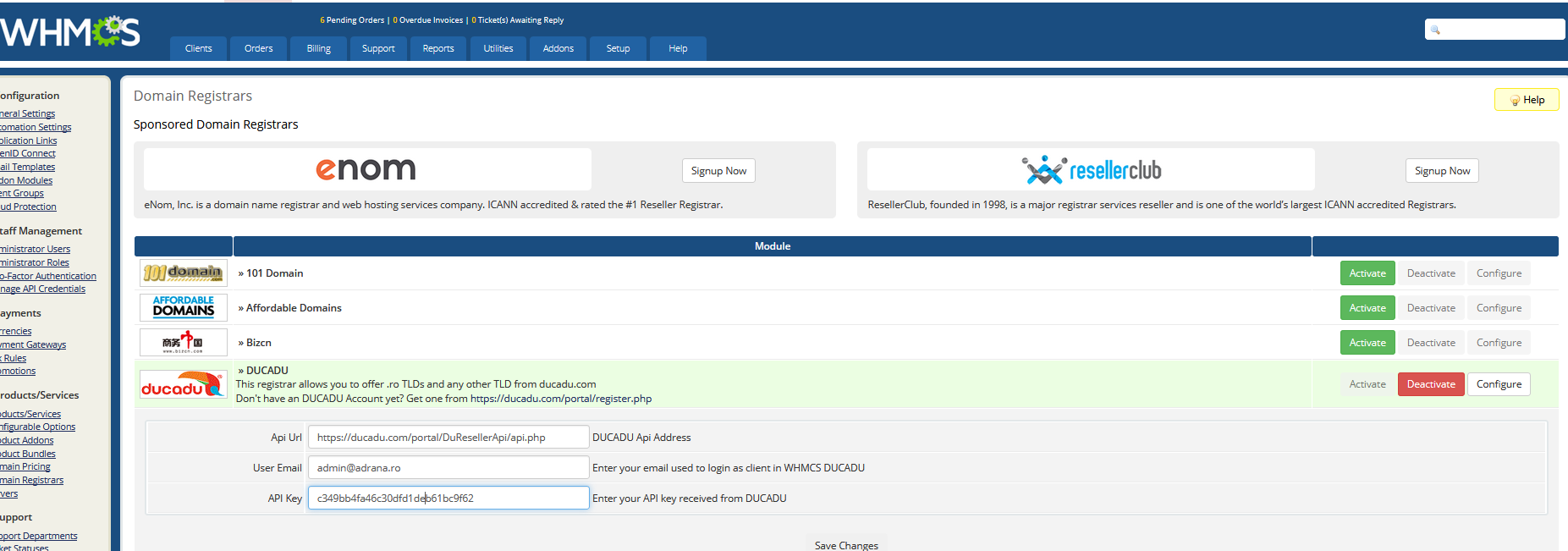This image captures a computer screenshot of a platform related to Enom and ResellerClub, specifically dealing with domain management through the WHMCS (Web Host Manager Complete Solution) interface. The title prominently features the term "Affordable Domains," indicating a focus on cost-effective domain registration services. The main section of the screenshot includes functionalities such as "Activate," "Deactivate," and "Configure" for domains, with a repeated emphasis on "101 Domains." These interactive buttons suggest options for managing domain status and settings. Additionally, there are mentions of an unfamiliar term "DUCADU" on the right-hand side, whose exact meaning is unclear from the context. The overall image suggests the user is accessing a tool for domain registration and management, although the specific details and usability elements might not be fully clear to those unfamiliar with domain and web hosting technologies.